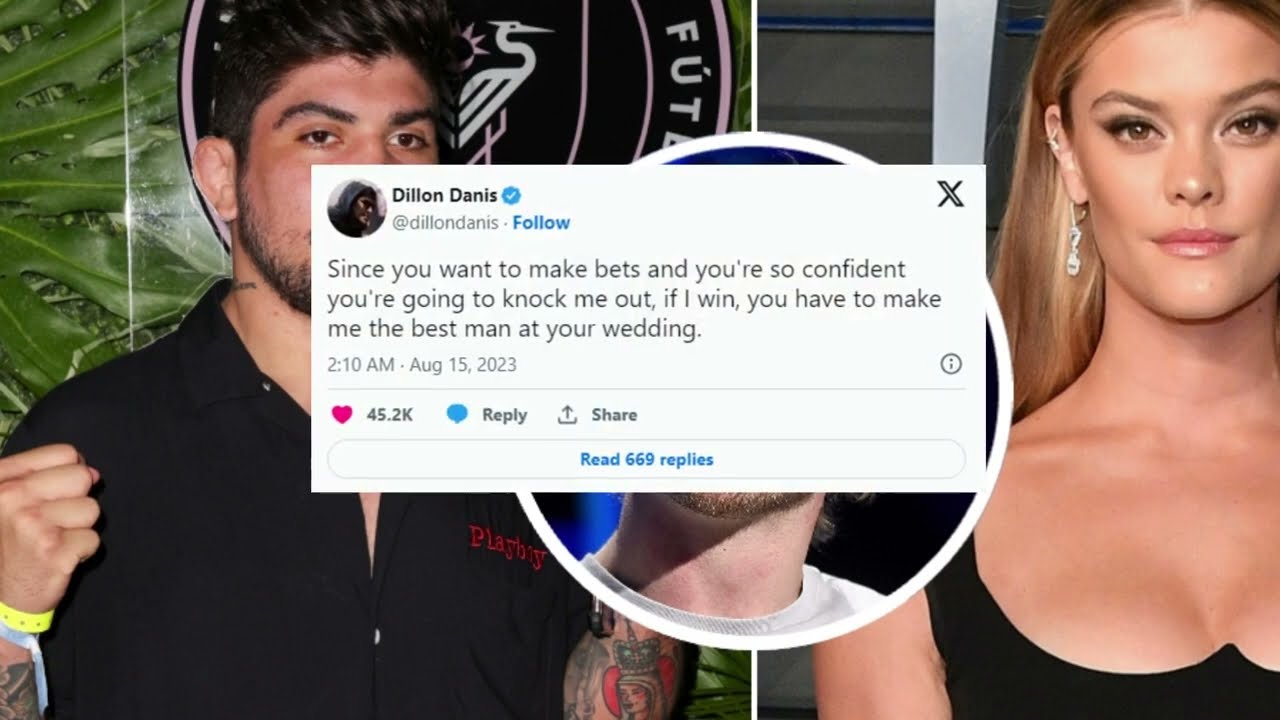This image features a tweet from the verified Twitter account of Dylan Danis (@DylanDanis) prominently displayed in the center, partially obscuring the background visuals. The tweet, timestamped at 2:10 AM on August 15, reads: "Since you want to make bets and you're so confident you're going to knock me out. If I win, you have to make me the best man at your wedding." Accompanying interaction details include 45.2K likes, a reply button with 669 replies, and a share icon.

Behind the tweet, the image showcases a woman and a man. The woman is positioned on the right side, with long blonde hair, light skin, and pink lips. She wears a black dress with a distinctive neckline that forms a point in the middle of her chest. She accessorizes with dangly diamond earrings. The man, situated on the left, sports a black button-up shirt with red text on the pocket that reads "Playboy." He features dark hair, styled and gelled, a black beard, and black eyebrows. His visible hand tattoos and groomed appearance contribute to his striking look. The visual composition is split with a line down the middle, and there's an occluded image of another person, likely Dylan Danis, partially hidden behind the tweet overlay, creating a layered and intricate portrayal.